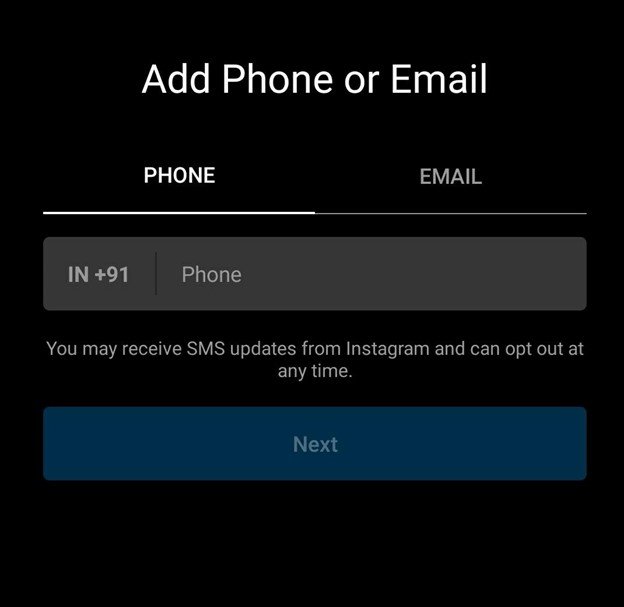The image features a large black square as the background. At the top center, in white text, it reads "ADD PHONE OR EMAIL." Below this, the word "PHONE" is displayed in uppercase white letters and is underlined with a white horizontal line. To the right, also underlined with a horizontal line but in light gray, is the word "EMAIL," spelled out as "E-M-A-I-L."

Further down, a gray rectangle contains the text "IN +91 | PHONE," indicating a placeholder for entering a phone number with the country code +91. Beneath this, in white text, there is a disclaimer: "YOU MAY RECEIVE SMS UPDATES FROM INSTAGRAM AND CAN OPT OUT AT ANY TIME," with "SMS UPDATES" in uppercase letters for emphasis.

At the bottom of the image, there is a long blue rectangle, and within it, the word "NEXT" is written in uppercase light blue letters. This marks the end of the described information.